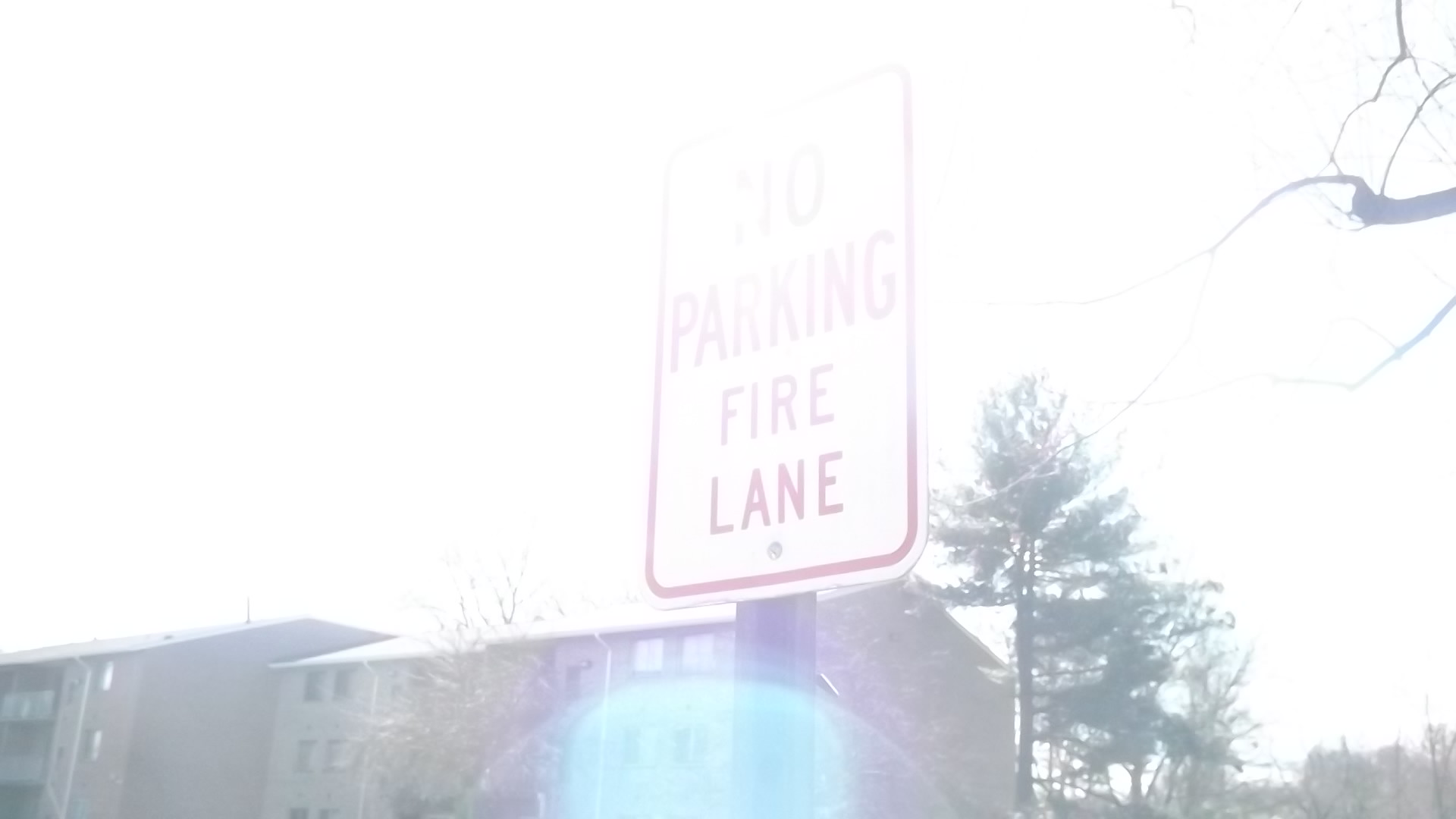In this highly overexposed photograph, taken with a digital camera or smartphone, the centerpiece is a white rectangular sign with red trim and red lettering that reads “No Parking, Fire Lane.” The sign is mounted on a dark-colored pole. Due to the significant backlight, the entire scene appears excessively bright, almost "whited out," making finer details difficult to discern. A noticeable lens flare in the form of a blue light sphere is visible toward the bottom of the image. In the background, two dark red brick apartment buildings with several stories and numerous windows stand prominently. These buildings feature balconies and are partially obscured by tall trees, including an evergreen to the side and another tree with bare branches in the upper right corner. The background elements suggest it’s an outdoor setting, likely in a residential or dormitory area.